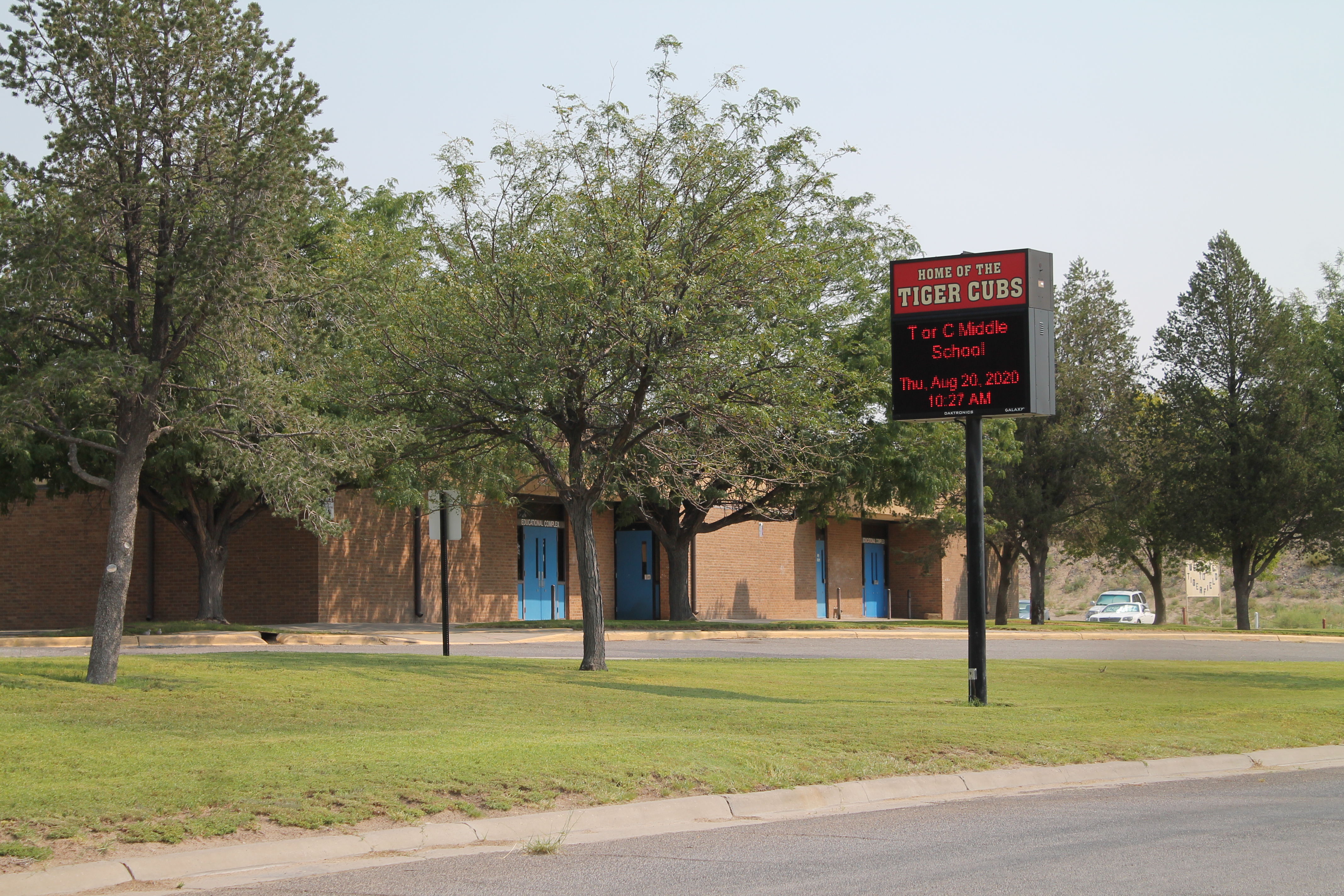This photograph captures the front of a one-story brick school building identified as T or C Middle School, home of the Tiger Cubs. The building features several blue metal entrance doors. Surrounding the school is a flat landscape with a well-maintained patch of short green grass in the foreground, bordered by a driveway or parking lot. Further back into the image, on the right side, you can spot a parking lot with a few cars, including at least one or two white vehicles. The background includes some deciduous trees, likely in full leaf suggesting the photo was taken in summer, partially obscuring distant hills. Prominently featured in the center of the image is a tall sign mounted on a black pole about 10 to 15 feet high. The sign, which is square and lit from within, has a red upper section displaying "Home of the Tiger Cubs" in white letters and a black section below with changeable orange digital lettering that reads "T or C Middle School" and shows the date and time: "Thursday August 20th, 2020, 10:27 a.m." There are no people visible, giving the school a quiet, inactive appearance, likely due to the summer break.